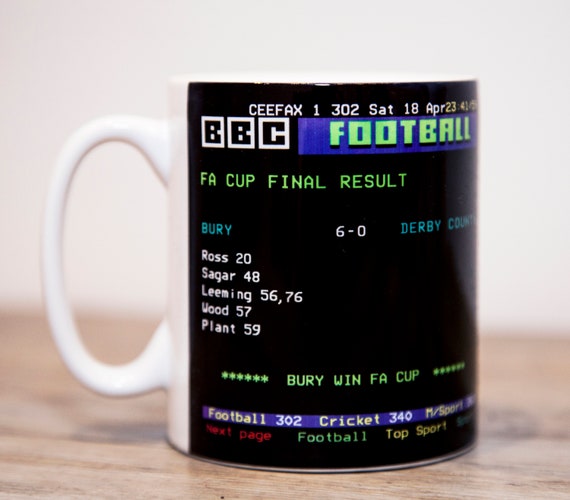This square image features a detailed close-up of a white coffee mug with a white handle positioned to the left, resting on a medium brown wooden surface with visible dark wood knots and grains. The background is divided, with the top half displaying a white or light gray wall, adding contrast to the scene. The front side of the mug showcases a black rectangular area designed to resemble a vintage sports scoreboard or digital display screen.

The top of the black rectangle on the mug prominently features the text "BBC FOOTBALL" with "BBC" printed in black letters inside of white squares, followed by "FOOTBALL" in block letters that are light green against a blue rectangular background. Below this, the text "FA CUP FINAL RESULTS" is printed in all caps green, followed by match details:

- BURY 6-0 DERBY COUNTY
- Scorers for Bury: ROSS (20'), SAGER (48'), LEEMING (56', 76'), WOOD (57'), PLANT (59')

At the bottom of this black area, a horizontal banner displays green stars with the text "BURY WIN FA CUP" interspersed between them, reinforcing the match outcome. The design elements use a variety of colors, including blue, black, white, and off-green, enhancing the retro aesthetic of the "screen."